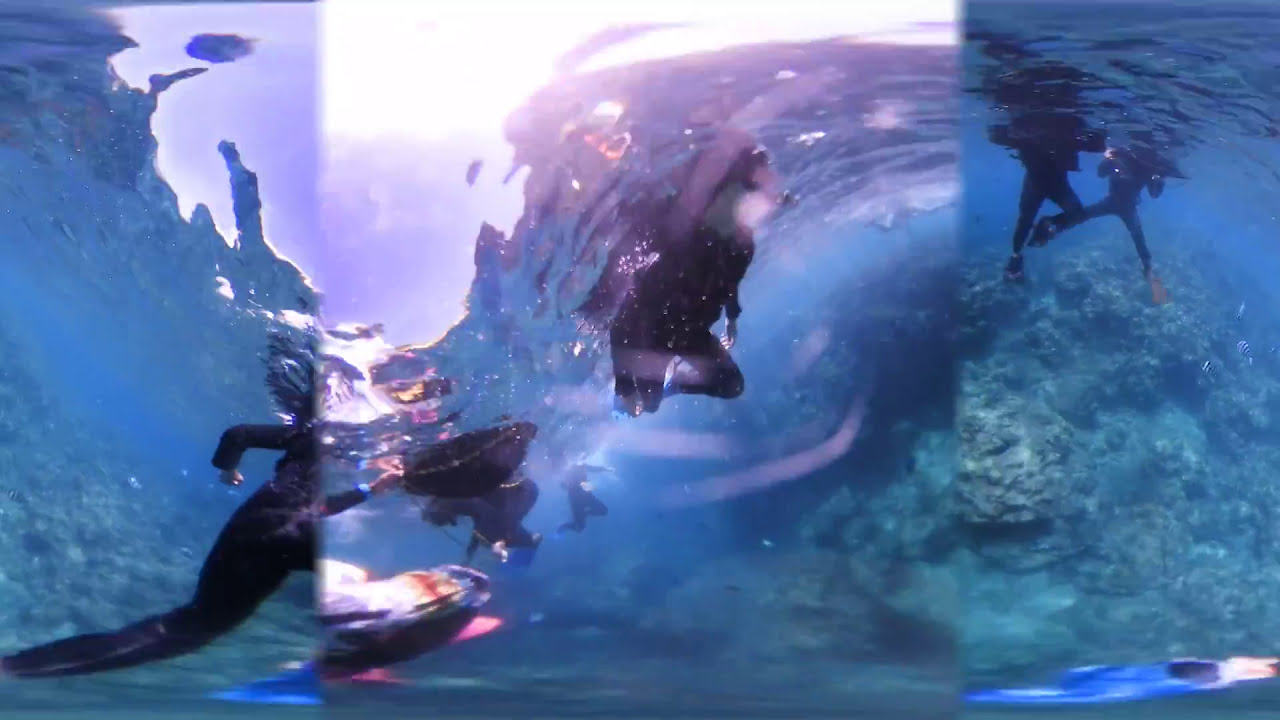This underwater photograph, likely taken with a scuba-safe camera, captures a serene and slightly distorted ocean scene with a vivid blue background. The image, horizontal and rectangular in format, features rippling water and the distinct presence of five scuba divers. They are all donned in black full-body diving suits, complete with fins, oxygen tanks on their backs, and face masks. 

In the lower left-hand corner, some fish can be seen swimming amid a flourishing collection of bluish-green algae. Moreover, the seafloor, dotted with gray and brown rocks and possibly some coral, comes into view as well. The composition also reveals a striking ray of sunlight piercing through the water, illuminating the center of the photograph and creating a lighter area among the divers. 

The divers are located in various positions: one on the left, one near the center, and two more visible in the upper right-hand corner, where their heads break through the surface. A fifth diver is also discernible, adding to the dynamic arrangement. Above, the waves are choppy, and you can see breaks in the waves, which contribute to the image’s overall feeling of a tranquil yet lively underwater world.